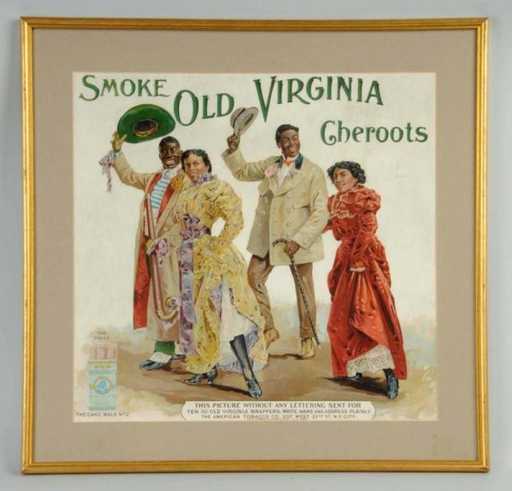This vintage cigarette advertisement, showcased within a thin, gold metal frame and mounted on a gray wall, displays an illustration beneath prominent green text that reads "Smoke Old Virginia Cheroots." The central image depicts two African-American couples dressed in 1700s or early 1800s attire. The men, wearing top hats—one green and one gray—hold their hats aloft in a friendly gesture while carrying canes. They are dressed in beige suit coats with one man donning a striped shirt and green pants beneath a red robe. The women, linked arm-in-arm with the men, wear ornate blouses and long dresses—one in flowing yellow with purple accents and the other in red. Displaying a slightly coquettish manner, the women lift the hems of their dresses to reveal their slips and ankles, adorned in high-heeled black leather boots. In the bottom left corner, a partially visible turquoise cigarette pack adds a subtle nod to the product being advertised. Additional small text at the bottom center is too diminutive to read clearly.